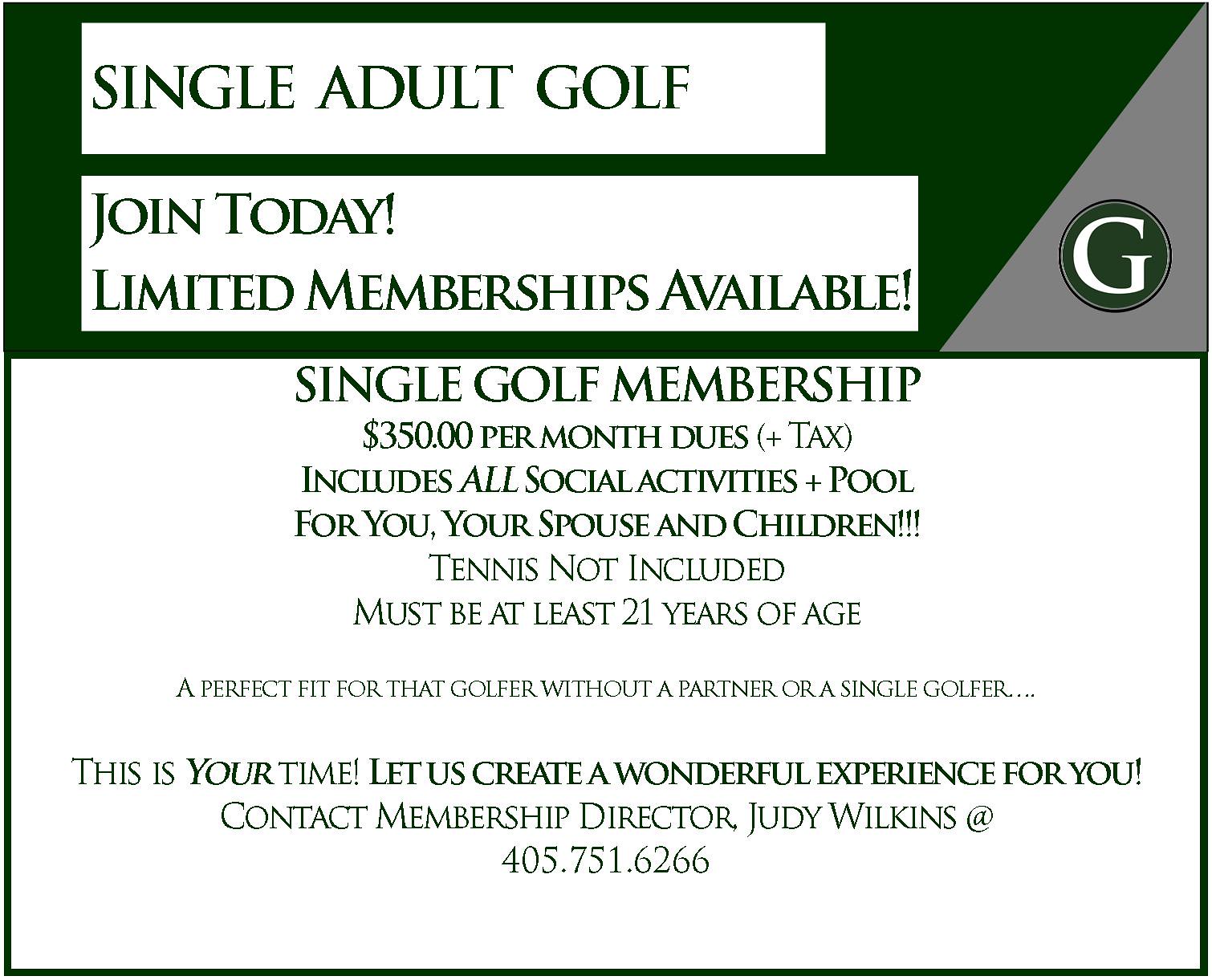The image is a predominantly green, gray, and white poster or presentation slide focusing on text. The black-and-white sign prominently displays "Single Adult Golf" at the top, encouraging viewers to "Join Today." It mentions "Limited memberships available" just below. The main section details a "Single Golf Membership" priced at $350 per month, plus tax. The membership includes all social activities and access to a pool for you, your spouse, and children, though tennis is not included. Eligibility requires members to be at least 21 years of age, making it an ideal option for single golfers. The promotional message emphasizes, "This is your time. Let us create a wonderful experience for you." For more information, viewers are directed to contact Membership Director Judy Wilkins at 405-751-2666. The text is well-spaced, enhancing readability in what appears to be an advertisement for a golf course.